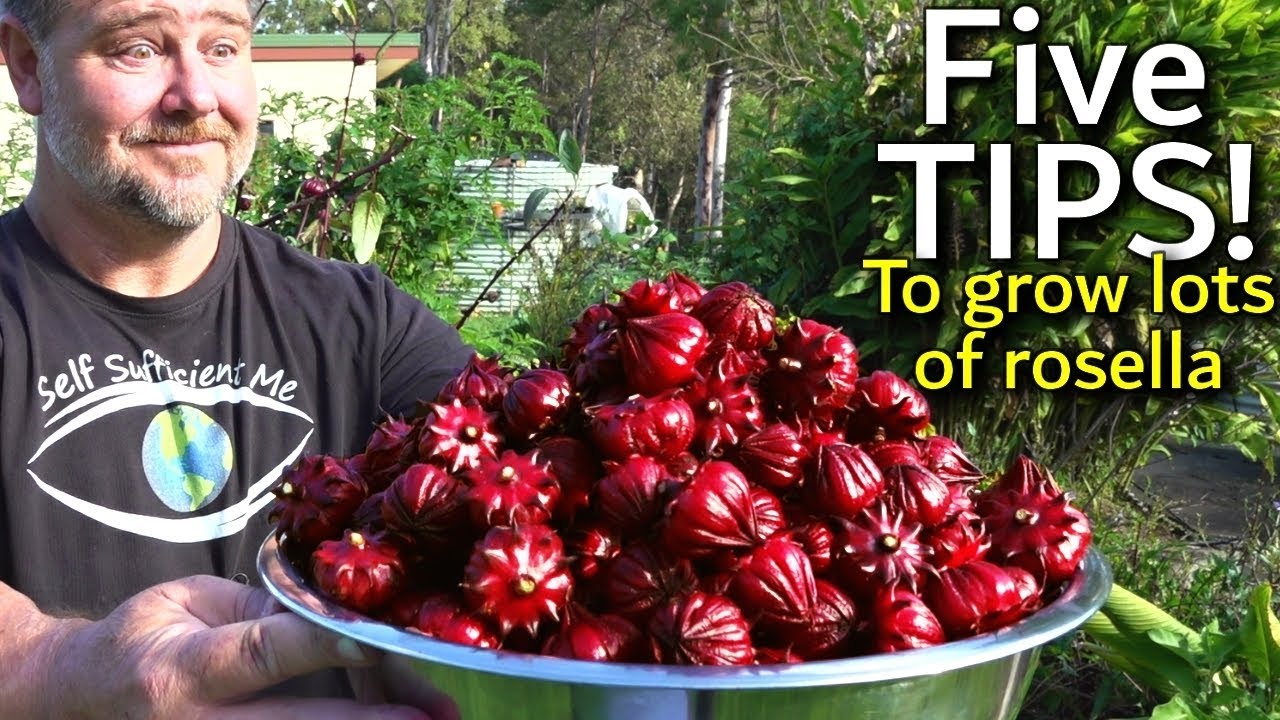The image is a YouTube thumbnail featuring a photograph with digitally added text in the top right corner. The text reads "5 tips!" in bright white font, followed by "to grow lots of Rosella" in yellow font, both with a black border. The main photograph shows a cheerful man, likely in a garden, holding a shiny metallic bowl filled with crimson, spiky fruits identified as Rosella. The man, wearing a black t-shirt that says "self-sufficient me" and featuring a unique eye-with-earth logo, sports a short beard and displays a pleasantly surprised expression. The lush green background complements the vibrant red fruits in the bowl.